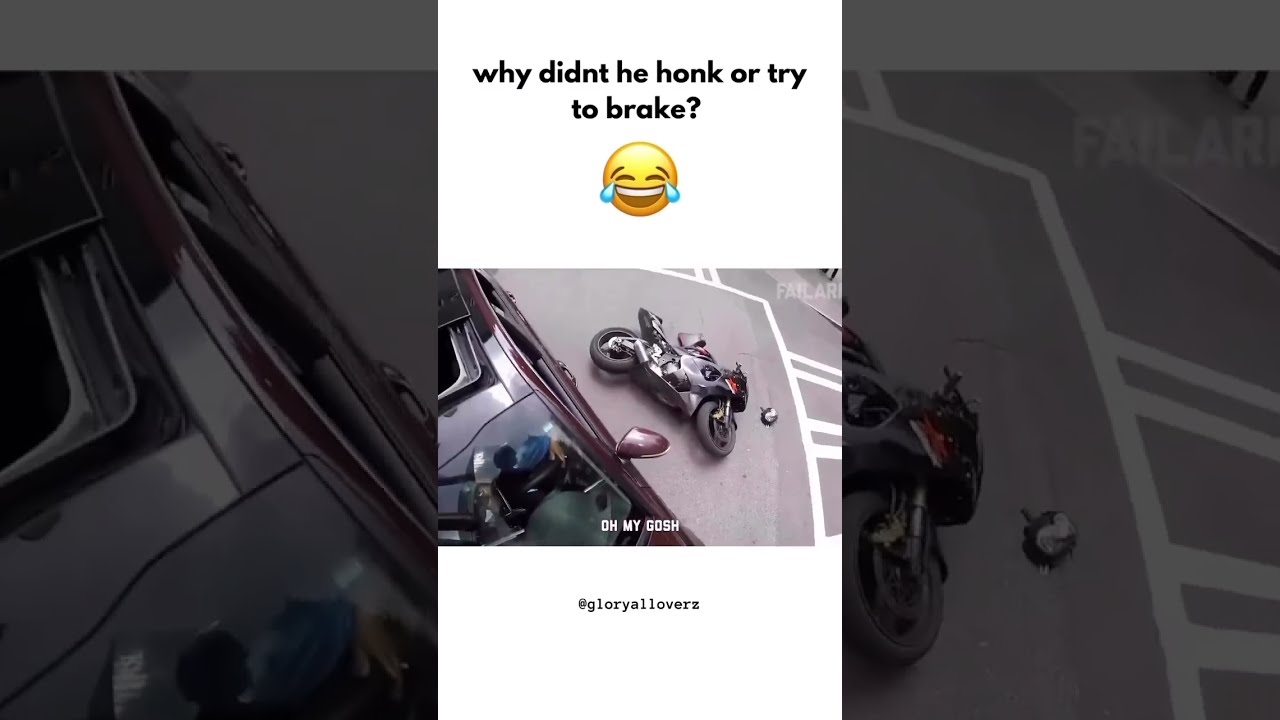The image is a composite of both photographic and computer-generated elements, presented in a horizontal rectangular format. At its center is a vertical rectangle showcasing a color photograph that appears as though it was taken with a cell phone, depicting a vivid and dramatic scene on gray asphalt with white markings. This central photograph features a purple SUV stopped on the road and a motorcycle lying on its side beside it. A broken piece of the motorcycle or scooter, possibly a helmet or equipment, lies nearby. Although it seems like there has been an accident, there are no visible injured individuals. Above the photograph, a meme headline reads in bold black text on a white background, "Why didn't he honk or try to brake?" followed by a crying-laughing emoji. Below the image is a caption in all caps white letters, stating, "Oh my gosh!" Further down, a hashtag "#gloryalloverz" appears in gray text.

Flanking this central photo are two grayed-out, black-and-white close-up panels that are enlarged sections of the same photograph. The left panel shows a close-up of the SUV, while the right panel displays part of the motorcycle lying on the road with a broken piece of its equipment. The contrasting detail between the color central image and its monochromatic side enlargements heightens the sense of focus and intensity on the main scene.